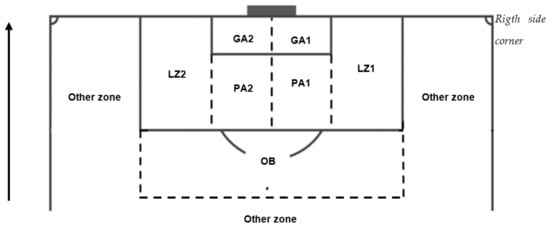This black-and-white blueprint-style design resembles a top-down view of a divided sports court, potentially a basketball half-court. The diagram is intricately labeled with alphanumeric codes and features a mixture of solid and dashed lines to demarcate various sections. An arrow on the far left side points upwards, guiding the orientation of the diagram.

On the upper right-hand side, a prominent rectangle spans the width and bears the label "right side corner." Adjacent to it, on the left, is an area marked "Other Zone." Within the expansive rectangle, there are multiple internal groups of rooms and zones separated by both dashed and solid lines. From left to right and top to bottom, these labeled sections include:

- "LZ2" in a vertically oriented rectangle
- "GA2" next to LZ2, separated by dashed lines
- "GA1" beneath GA2, and separated by another solid line
- Further down are "PA2" and "PA1," each compartmentalized by dashed lines
- "LZ1," situated below PA1, is demarcated by a solid line before transitioning into another section termed "Other Zone."

An additional checked-off area within the diagram shows dashed boundaries and carries the labels "Other Zone" on one side and "OB" on the opposite side. This detailed plan conveys distinct spatial divisions and labeled zones, creating an organized and comprehensible layout of what appears to be a sports facility's partial blueprint.